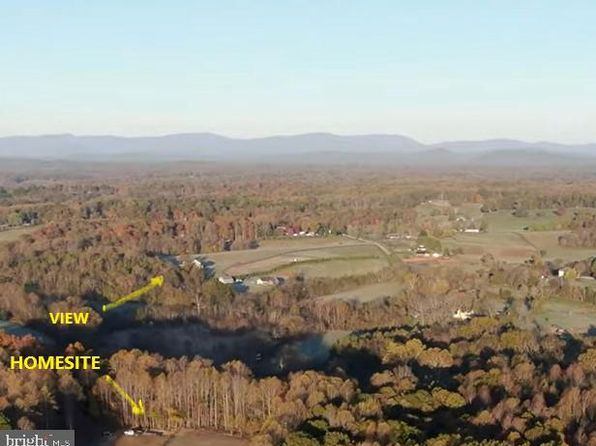The image captures a rural setting from an overhead or bird's eye perspective, likely showcasing real estate property. In the immediate foreground toward the left, there are labels in yellow text; one reads "home site" with an arrow pointing downward, indicating the location of the property. Behind this is another label that says "view" with an arrow pointing toward the scenic background. The scenery features a brownish landscape with several structures and buildings dispersed across large plots of land, interspersed with a lot of trees, plants, and bushes. The right side of the image includes open fields or farmland. In the distance, the shot captures a blue sky and a majestic mountain range. Additionally, at the bottom left corner, there's a watermark reading "Bright LMS," likely associated with the real estate entity "Bright Homes." Altogether, this detailed shot highlights the expansive and picturesque nature of the rural property and its surroundings.